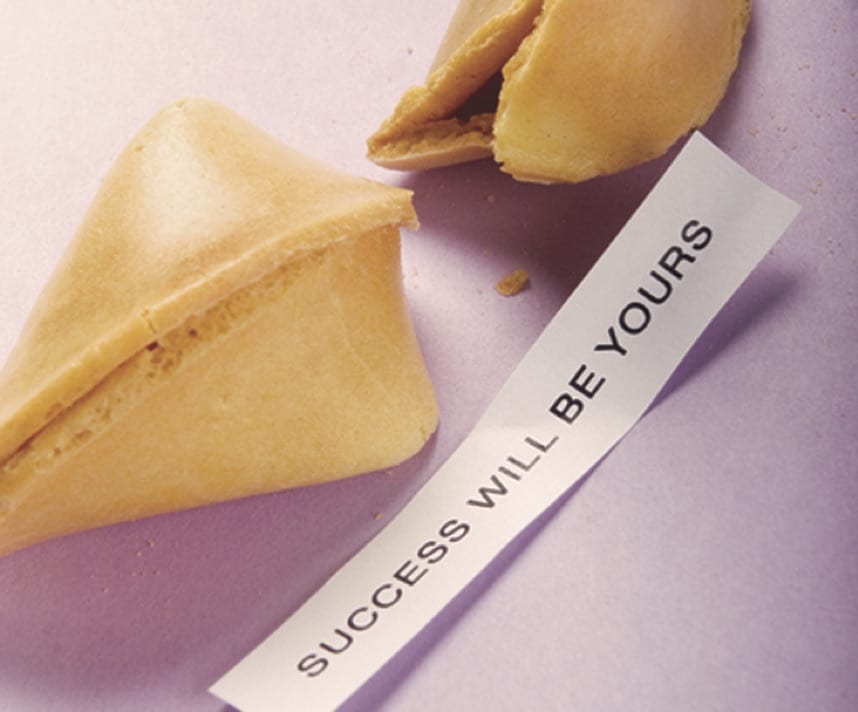This close-up photograph, set against a slightly purplish pink background, features two tan-colored fortune cookies diagonally arranged from the lower left to the top right. The cookie on the left displays its full seam, while the right cookie lies on its side, slightly open where the fortune has been removed. Scattered between the cookies are tiny crumbs and a broken piece, likely fallen from the open cookie. The fortune, reading "Success will be yours" in black capital letters, lies diagonally across a white strip from the bottom left to the top right. The image, illuminated from the top left, captures shadows from the fortune cookies and the paper strip, enhancing the photo's realism and detail.